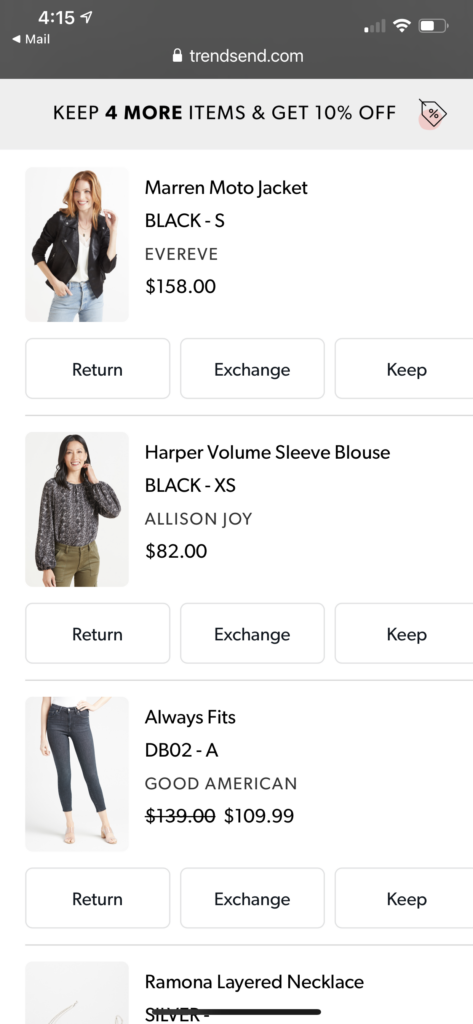The screenshot features a mobile shopping app interface with various clothing items and shopper options. At the top, there is a black status bar displaying the time as 4:15, a lock icon from the website transcend.com, one out of four signal bars, approximately half a battery life, and a Wi-Fi signal. Below this, a promotional message reads, "Keep four more items and get 10% off."

The main portion of the screen shows several pieces of clothing with images and detailed descriptions:

1. An image of a woman wearing a black jacket is accompanied by the following details: "Marimoto Jacket, Black - S, EverEve, $158." Below this, there are three buttons labeled: "Return," "Change," and "Keep."

2. A woman modeling a long-sleeve blouse with jeans is described with: "Harper Volume Sleeve Blouse, Black - XS, Alice and Joy, $82." Similarly, beneath this image, there are also "Return," "Change," and "Keep" buttons.

3. Another section showcases someone in blue jeans, labeled: "Always Fits, DV02 - A, Good American, $109.99."

Each item is presented clearly, allowing the viewer to decide whether to return, change, or keep each piece using the respective buttons situated below their descriptions.